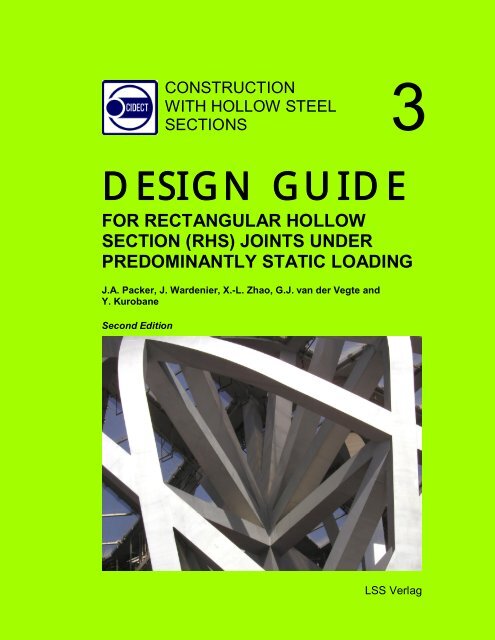The image depicts a design guide poster with a vivid lime green background. At the top, the poster features an insignia and the text "Construction with Hollow Steel Sections" prominently, accompanied by a large number "3" to its right. Below this, the title "Design Guide for Rectangular Hollow Section (RHS) Joints Under Predominantly Static Loading" is displayed in bold black letters. The authors listed are J. A. Packer, J. Wardenier, X. L. Zhao, G. J. Van Der Vegte, and Y. Kurumbane, followed by the notation "Second Edition." Central to the poster is an image of metal bars arranged in a crisscross pattern, suggesting construction elements, with the bars appearing to be both rectangular and hollow. The overall layout and the repeated emphasis on specific details imply this is a comprehensive guide related to construction and engineering.